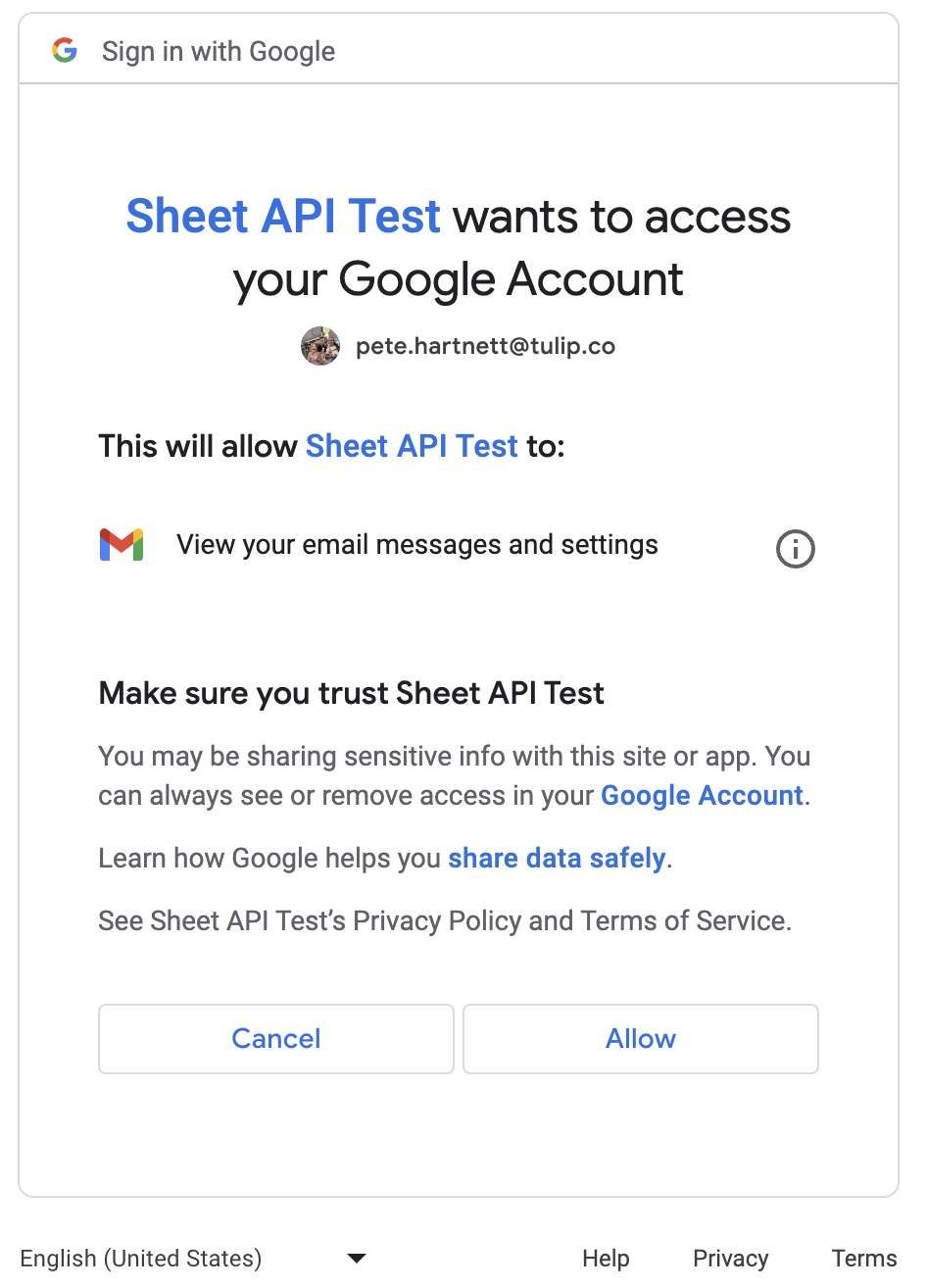The image depicts a computer notification requesting the user to sign in with their Google account. The notice specifies that "Sheet API Test" wishes to access the user's Google account, identified as peat.heartnett@tulip.com. Tulip is specified as the flower. It states that granting permission will enable "Sheet API Test" to view email messages and settings. A cautionary note reminds the user to trust "Sheet API Test" before proceeding, as sharing sensitive information with this site or app is possible. The notification also reassures that users can always see or remove access through their Google account settings, with the phrase highlighted as a clickable link. Additional links to learn how Google helps in safely sharing data, along with the "Sheet API Test" privacy policy and terms of service, are provided. The prompt concludes with two buttons, "Cancel" and "Allow," and a reference to www.google.com for more information.